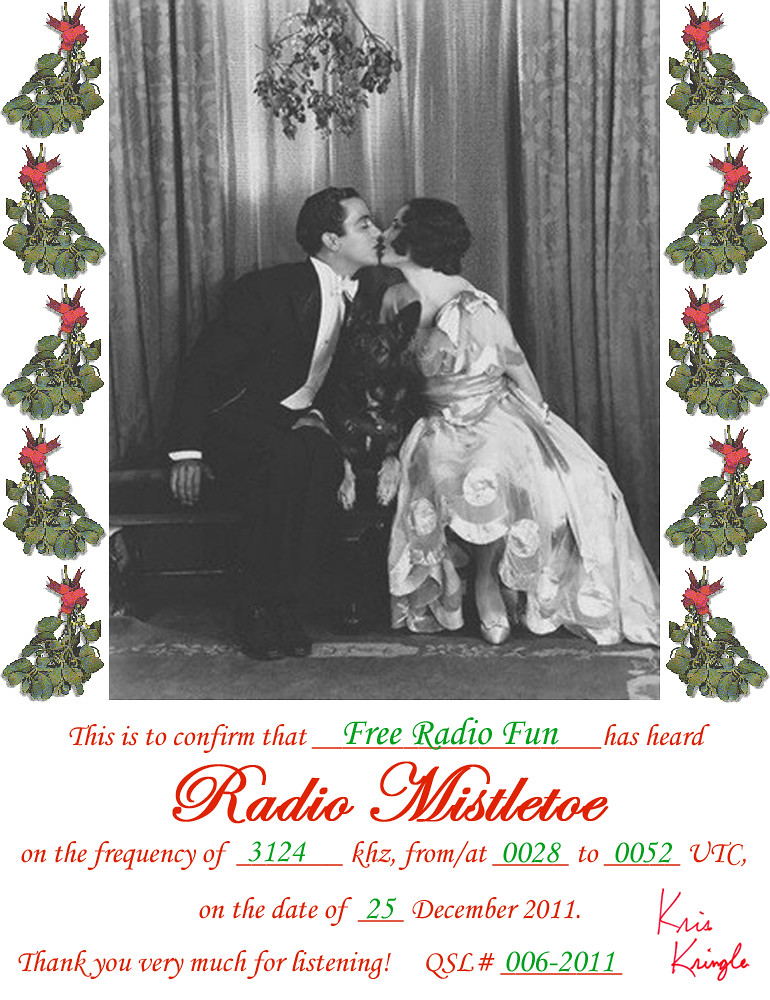The image showcases a vintage-themed event flyer featuring a central black-and-white photograph reminiscent of early 20th-century cinematography. The photograph captures a couple, a man in a suit and a woman in a formal dress, almost kissing while seated on a bench, with a German shepherd nestled between them. This romantic scene is framed by illustrations of mistletoe on both the left and right sides. Below the photograph, red and green text reads: "This is to confirm that Free Radio Fun has heard 'Radio Mistletoe' on the frequency of 3124 kHz from 0028 to 0052 UTC on the date of 25 December 2011. Thank you very much for listening. QSL number 006-2011." The confirmation is signed by Chris Kringle. The entire flyer adopts a vertical rectangular format, with the photograph positioned at the top and the festive-themed textual confirmation beneath it.